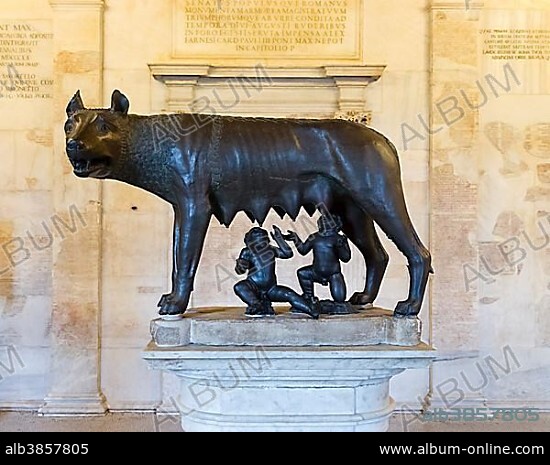The image depicts a detailed bronze statue of a large female wolf-like creature, possibly a hyena or dog, with eight prominent conical teats on its underside. The wolf stands on all four legs and is turned towards the left, glancing back towards the camera. Beneath the wolf, two human-like babies are depicted in positions of suckling from its teats—one sitting on its bum while the other is on one knee. The statue is mounted on a light gray stone pedestal and base. In the background, there is a light gray stone wall with columns and various inscriptions, although the text is too blurred to be legible. The image is watermarked with the word "ALBUM" repeated throughout, and in the bottom corners, it bears the text "ALB 3857805" on the left and "www.album-online.com" on the right. The overall setting is clear and brightly illuminated, likely due to natural light.